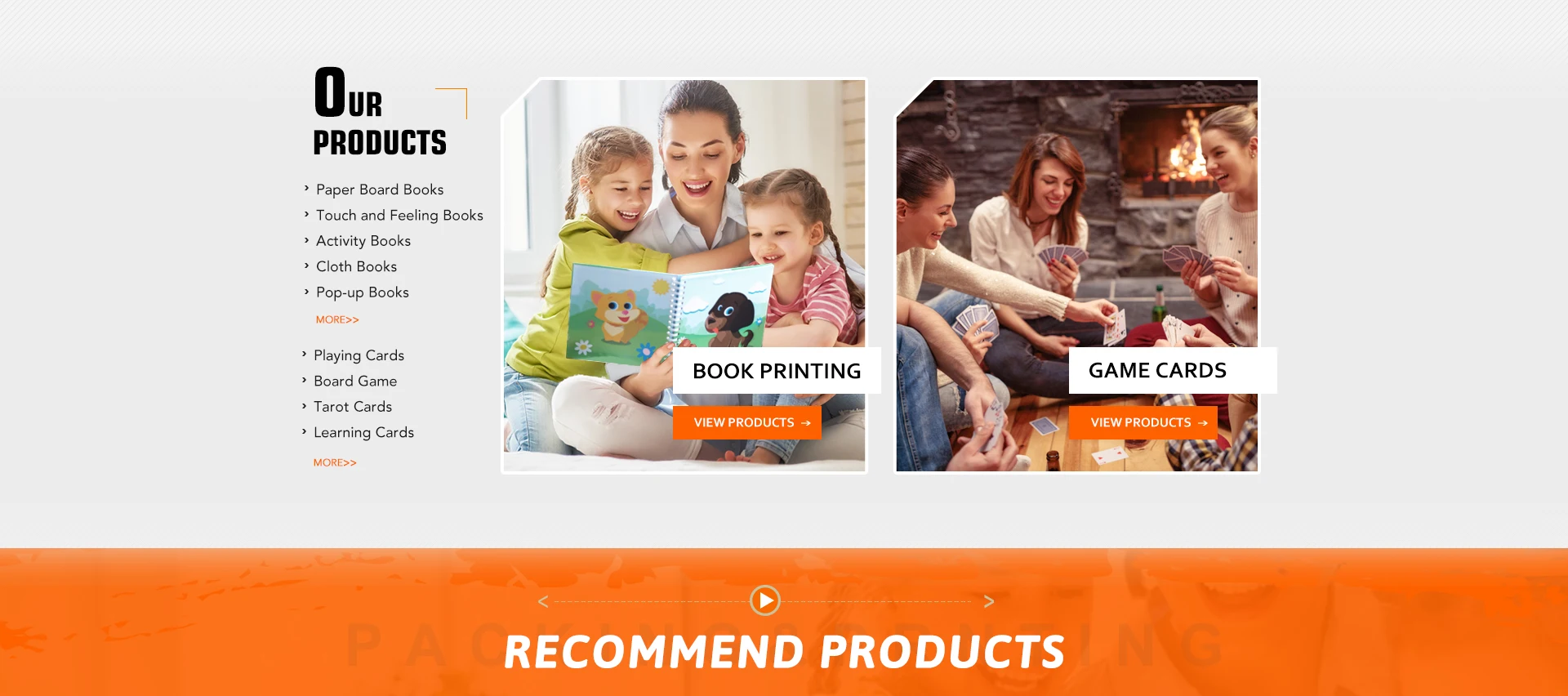The image, sourced from a website, features a top section with a light gray background and a wide orange strip at the bottom. Prominently displayed at the top is the heading "Our Products," followed by right-pointing arrows accompanied by labeled categories which are clickable. The categories listed include:

1. "Paper, Board, Books"
2. "Touch and Feeling Books"
3. "Activity Books"
4. "Cloth Books"
5. "Pop-Up Books"
   
Beneath these, there is an orange label "More" with two right-pointing arrows.

Further down, additional clickable categories are presented, including:

1. "Playing Cards"
2. "Board Game"
3. "Tarot Cards"
4. "Learning Cards"
   
This section also includes an area labeled "More," directing to further options.

In the middle of the image, two photographs are prominently displayed:
- On the left, a woman is reading a spring-bound book with animal illustrations to two smiling young girls sitting on her lap. This section is captioned "Book Printing" with a call-to-action "View Products."
- On the right, a group of women are depicted playing cards, with smiles all around and a cozy fire in the background. This section is labeled "Game Cards" with the same call-to-action, "View Products."

The bottom orange strip of the image contains the label "Recommend Products," drawing attention to suggested items.